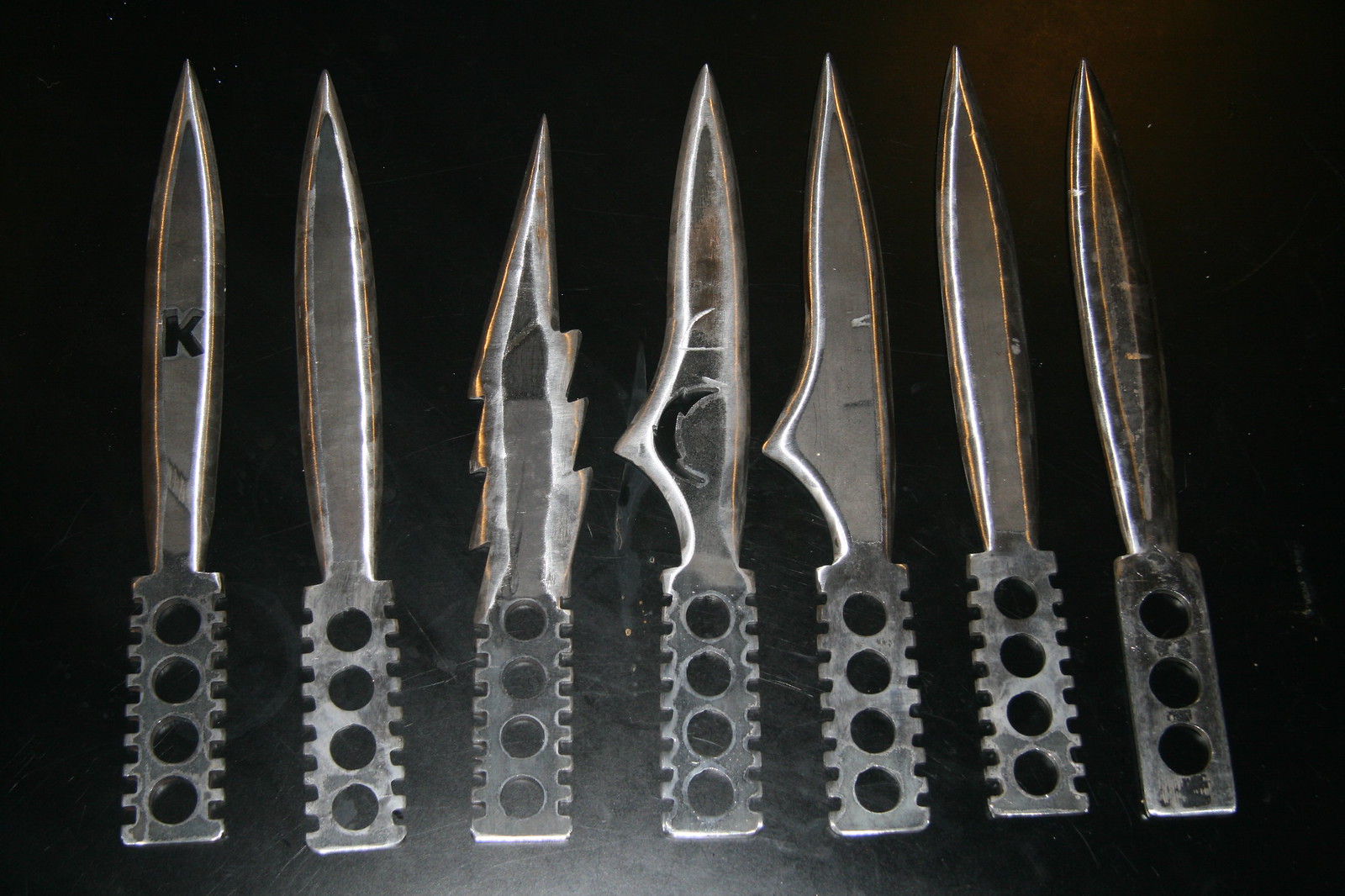This image is a detailed and realistic photograph of seven stainless steel knives laid out horizontally on a smooth, black surface, which could be plastic or metal. The knives are positioned with their blades pointing upwards and handles at the bottom. Each knife varies slightly in design but they all share some common features.

Starting from the left, the first knife is a sharp, serrated blade with the letter 'K' cut out and four holes in the handle area, presumably for grip. The second knife is similar in size and shape to the first but lacks any writing. It also has four holes in the handle section. The third knife is shorter with multiple jagged points jutting out from the blade. The fourth and fifth knives each feature a single serrated edge protruding to the left. The sixth knife closely resembles the second one, characterized by its straight edge and uniform holes. Lastly, the seventh knife on the far right is straight-edged with a pointed tip and three handle holes instead of four.

All knives are meticulously arranged side by side, creating a striking visual contrast against the deep black background. Their sleek, metallic surfaces gleam under the light, emphasizing their stainless steel material.